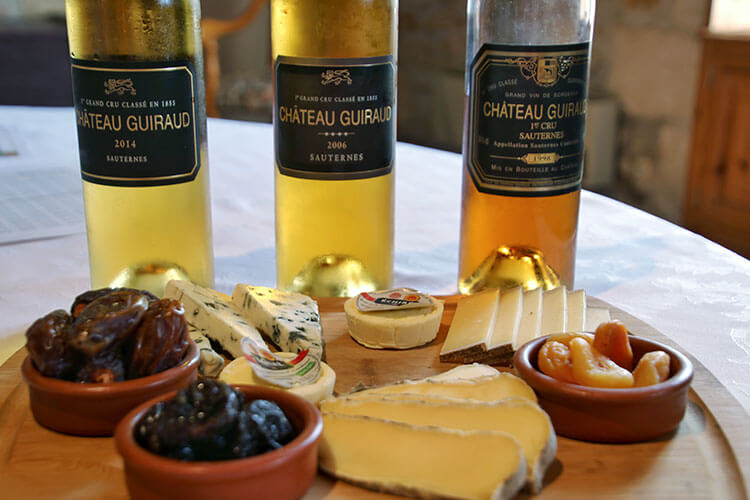The photograph features an elegant wine tasting setup on a white, rounded marble table set against a background with an out-of-focus exposed stone wall and some woodwork. The focal point of the image is a wooden rectangular platter laid with an array of cheeses and dried fruits, positioned in front of three glass bottles of Chateau Grand white wines. The cheeses are diverse, including soft cheese with blue specks, sliced cheeses, and a couple of small cheese wheels still wrapped with their labels. The dried fruits consist of dark brown dates, black prunes, and golden apricots, carefully placed in small clay crock containers. The three wine bottles stand in a row behind the wooden platter, with labels in black and gold font identifying them as Chateau Giraud wines from the years 2014, 2006, and possibly 1994. The leftmost and center bottles are full, while the rightmost bottle is half-full. This meticulously arranged tableau captures the essence of a sophisticated wine and cheese tasting experience.